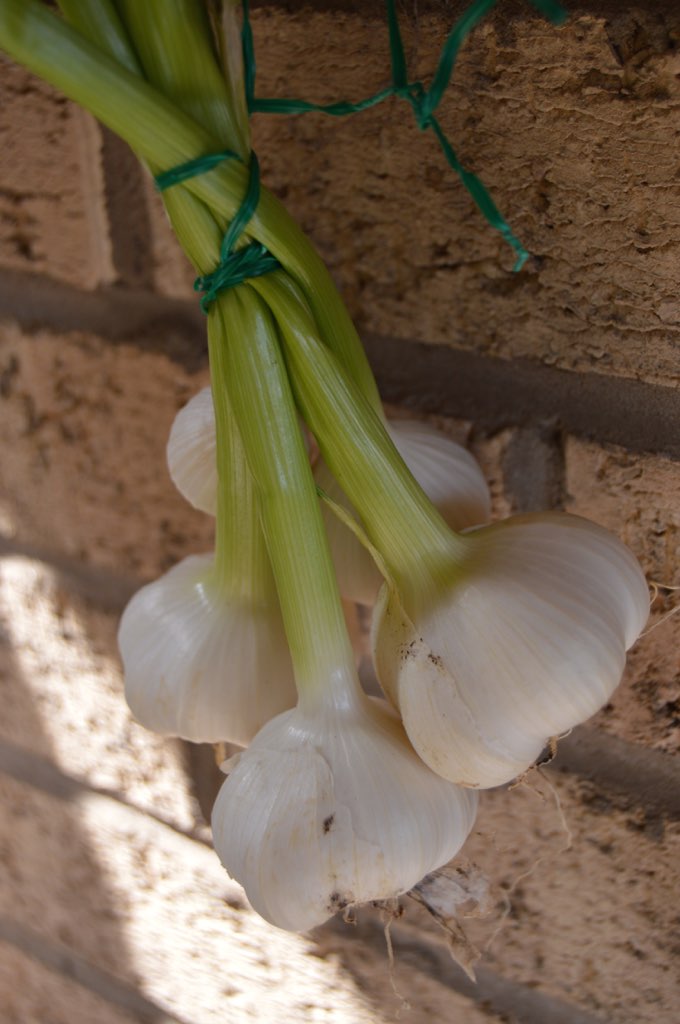This is a detailed close-up color photograph of a fresh bundle of garlic hanging upside down against a brown brick wall. The bundle consists of five garlic bulbs, with their long, light green stems, or chives, still attached. The garlic appears to have been recently pulled from the ground, as remnants of roots and traces of dirt are still visible on two of the bulbs. The garlic heads are tied together using a green twist tie, which secures them neatly. The white, fluffy garlic bulbs contrast against the brick background. The image, shot in portrait mode, includes a shaft of sunlight streaming in from the left corner, highlighting the health and freshness of the vegetables. There are no additional elements such as people, animals, or mechanical objects present in the composition.